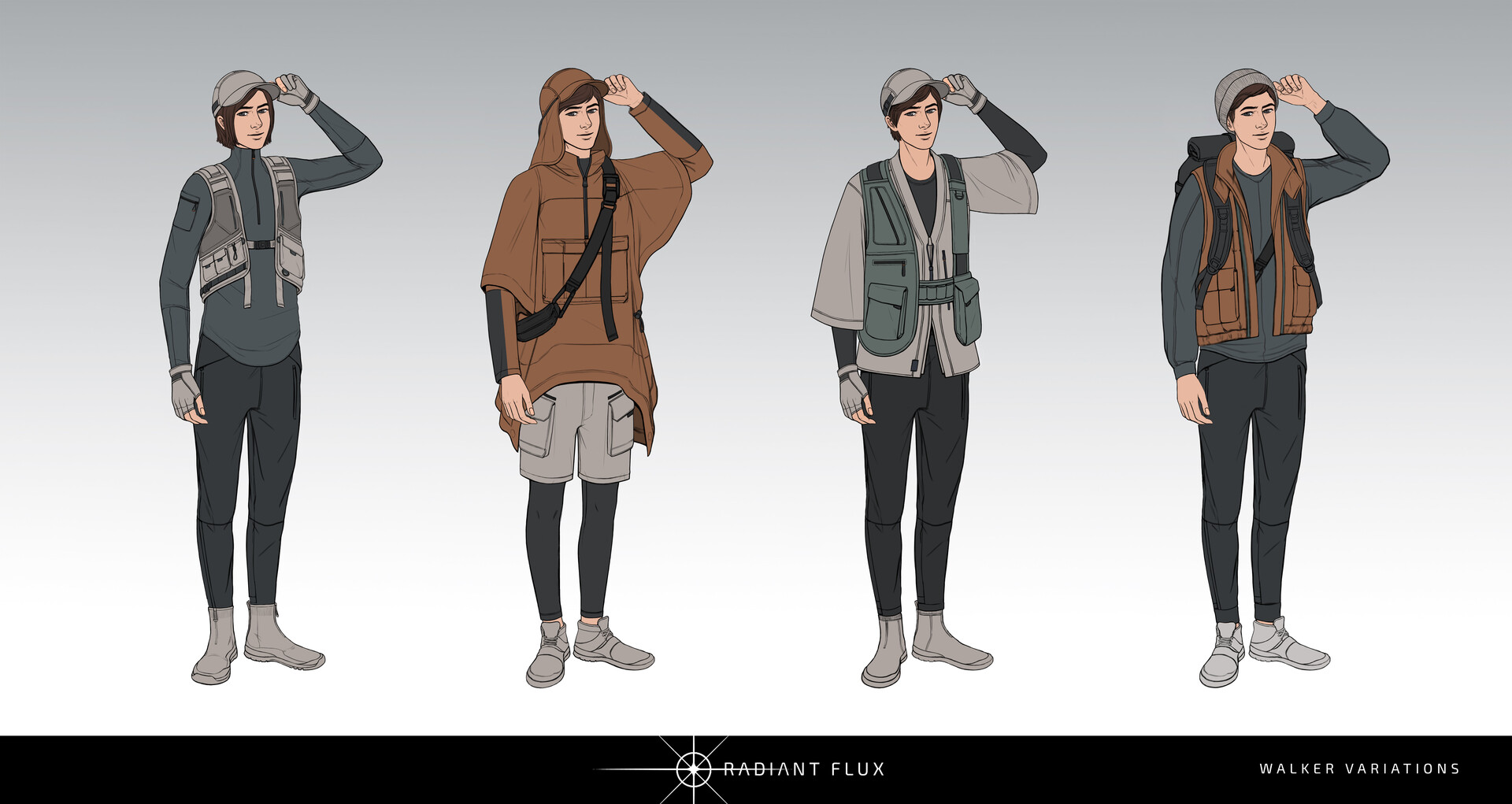The image is a digital, anime-style drawing depicting a tall, young white man with short brown hair, presented in four different outfits against a gray-to-white gradient background. A black stripe at the bottom right reads "Radiant Flux" alongside its logo, and the text "Walker Variations" appears on the right side of the image. Each variation of the man, who appears to be in his 20s, exhibits a distinct look focused on hiking gear and earth-toned clothing.

From left to right:

1. The first version shows him in a gray shirt, a vest, black pants, gray boots, a gray baseball cap, and gray fingerless gloves.
2. The second version features him in a brown poncho with a flap-back baseball cap, gray shorts over black leggings, and the same gray boots and fingerless gloves.
3. In the third depiction, he wears a gray loose top, a vest with pockets over a darker gray jacket, black pants, and a gray baseball cap, maintaining his gray boots and fingerless gloves.
4. The rightmost version displays him in a slightly puffy green top under a brown vest, a gray beanie, a black backpack, black pants, and gray fingerless gloves.

Each outfit showcases different elements of outdoor attire suited for hiking or walking.